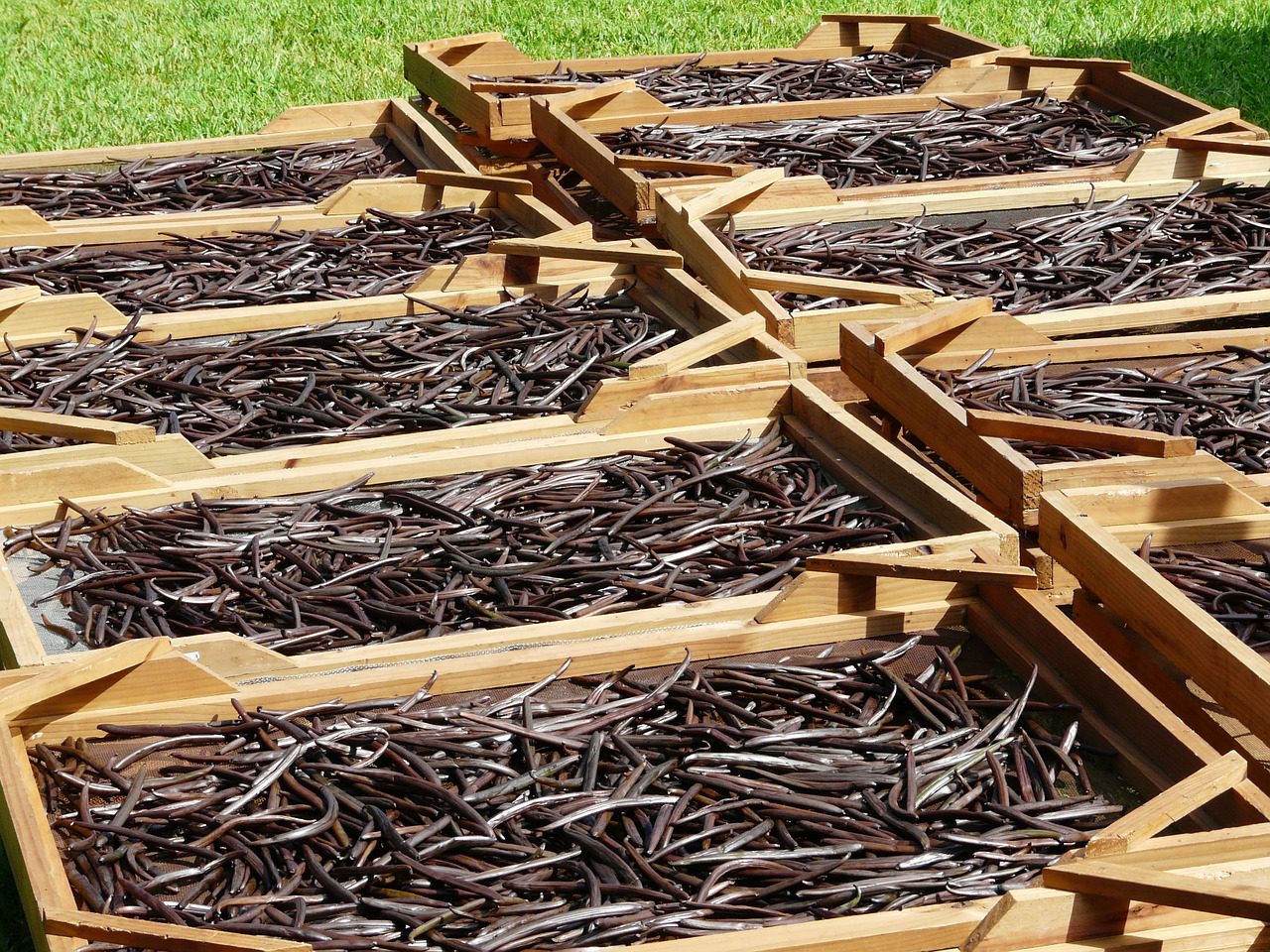The image features two parallel columns of rectangular wooden crates, possibly light golden or tan in color. Each crate includes angled slats diagonally across the corners, possibly serving as a lid mechanism or support. The crates are relatively thin and shallow, lined up neatly with some crates stacked one on top of the other. Inside each crate, there are numerous long, slender objects varying in appearance. Some of these objects are straight, while others are bent or curved.

The majority of the content appears metallic: some pieces are shiny and silver, catching the light, while others are dull and rusted, displaying a brownish hue. This gives the impression of various scraps or pieces of metal. Alongside the metallic elements, there are also descriptions that suggest the presence of organic material, such as vanilla beans or eel-like figures, displaying a brownish-gray color that is shiny, almost giving a slimy appearance.

All these crates are placed on a backdrop of freshly cut green grass, adding a contrast to the earthy and metallic tones of what's inside. This mixture of interpretations adds a unique and diverse visual texture to the scene.